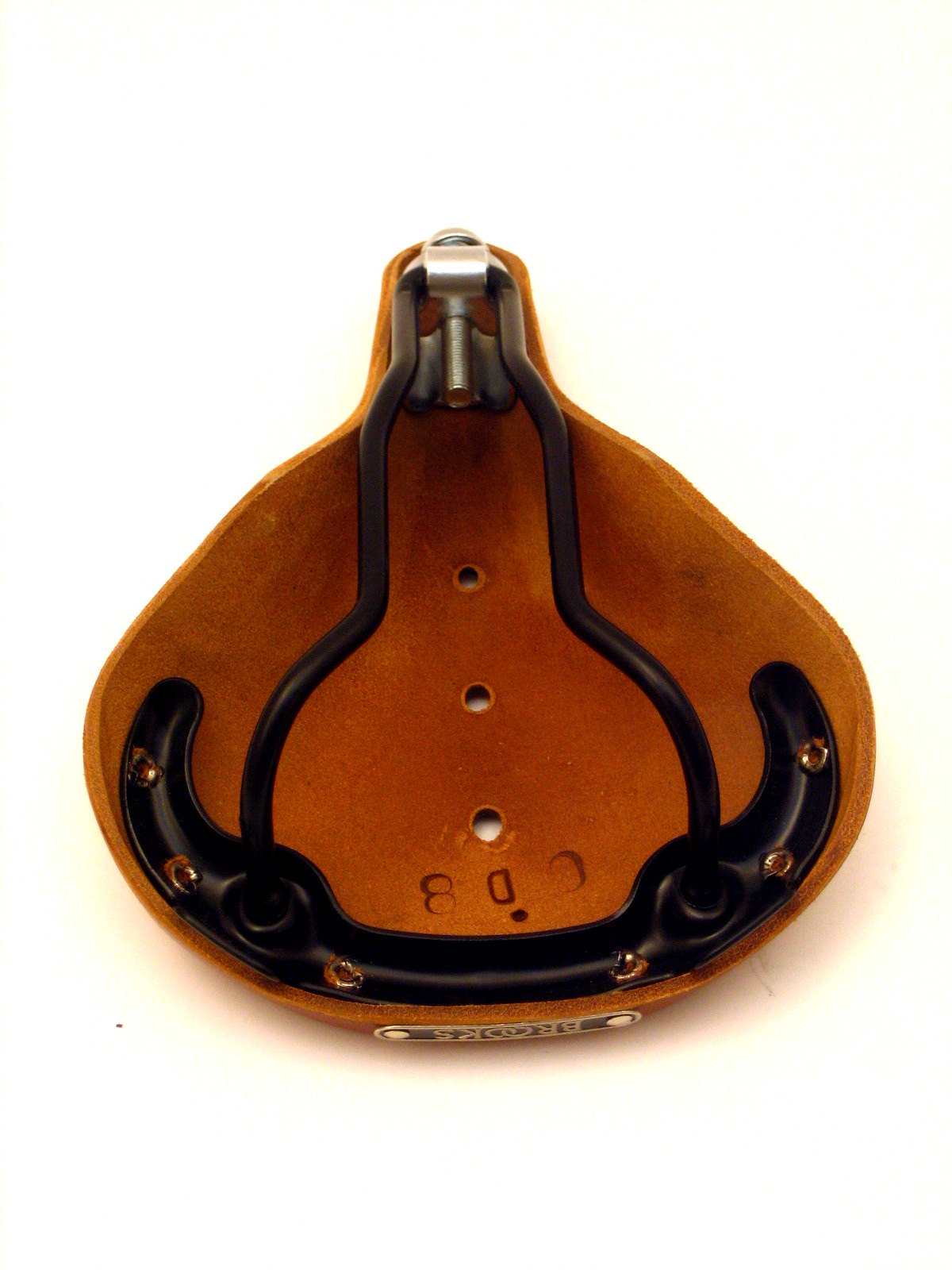The image depicts an upside-down bicycle seat positioned against a stark white background. The seat itself is a dark tan or brown color, with black metal bars forming a supportive frame underneath. Attached to the metal frame is a steel fastener and a small bell-shaped component, securing the frame and adding structural integrity. The back of the seat features a gold plaque, fastened with metal screws, although its inscription is unclear. In the middle of the seat are three small punch holes. Also visible are the upside-down letters "OD8" (alternatively "CD8"), which are likely branded markings on the seat. The captured perspective showcases the underside of the seat, emphasizing its robust construction and detailed components.